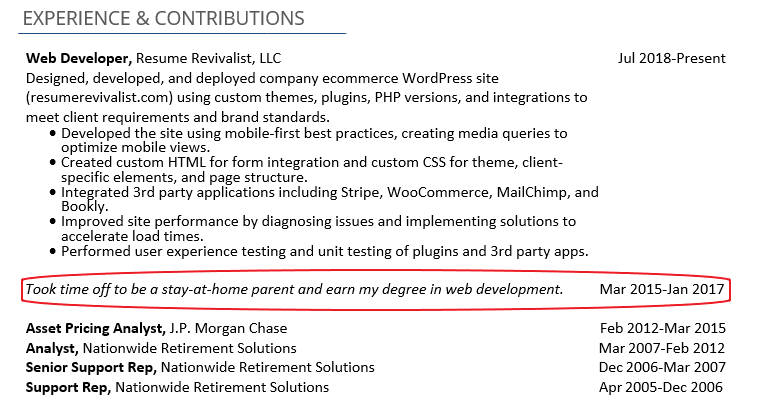Certainly! Here's a detailed and cleaned-up caption for the described image:

---

The image depicts a resume page focused on professional experience and contributions. At the top, the header "Experience and Contributions" is prominently displayed with a blue underline. Below this header, in black text, the position "Web Developer" at "Resume Revivalist LLC" is listed. This section details various responsibilities and achievements, including the design, development, and deployment of the company’s eCommerce WordPress site (ResumeRevivalist.com). Key tasks outlined include utilizing custom themes, plugins, and PHP versions to meet client requirements and brand standards, employing mobile-first best practices with media queries for optimal mobile views, and creating custom HTML for form integration and custom CSS for client-specific elements and page structures. Additionally, the role involved integrating third-party applications like Stripe, WooCommerce, MailChimp, and Bookly, improving site performance by diagnosing issues and accelerating load times, as well as performing user experience testing and unit testing of plugins and third-party apps.

A red circle highlights a note that says, "Took time off to be a stay-at-home parent and earned my degree in web development, March 2015 to January 2017."

Below this section are chronological details of other resume entries:
- **Asset Pricing Management, JPMorgan Chase:** February 2012 to March 2015
- **Analyst, Nationwide Retirement Solutions:** March 2007 through February 2012
- **Senior Support Rep, Nationwide Retirement Solutions:** December 2006 through March 2007
- **Support Rep, Nationwide Retirement Solutions:** April 2005 through December 2006

The entire content is presented on a clean white background with black text, ensuring readability and professionalism.

---